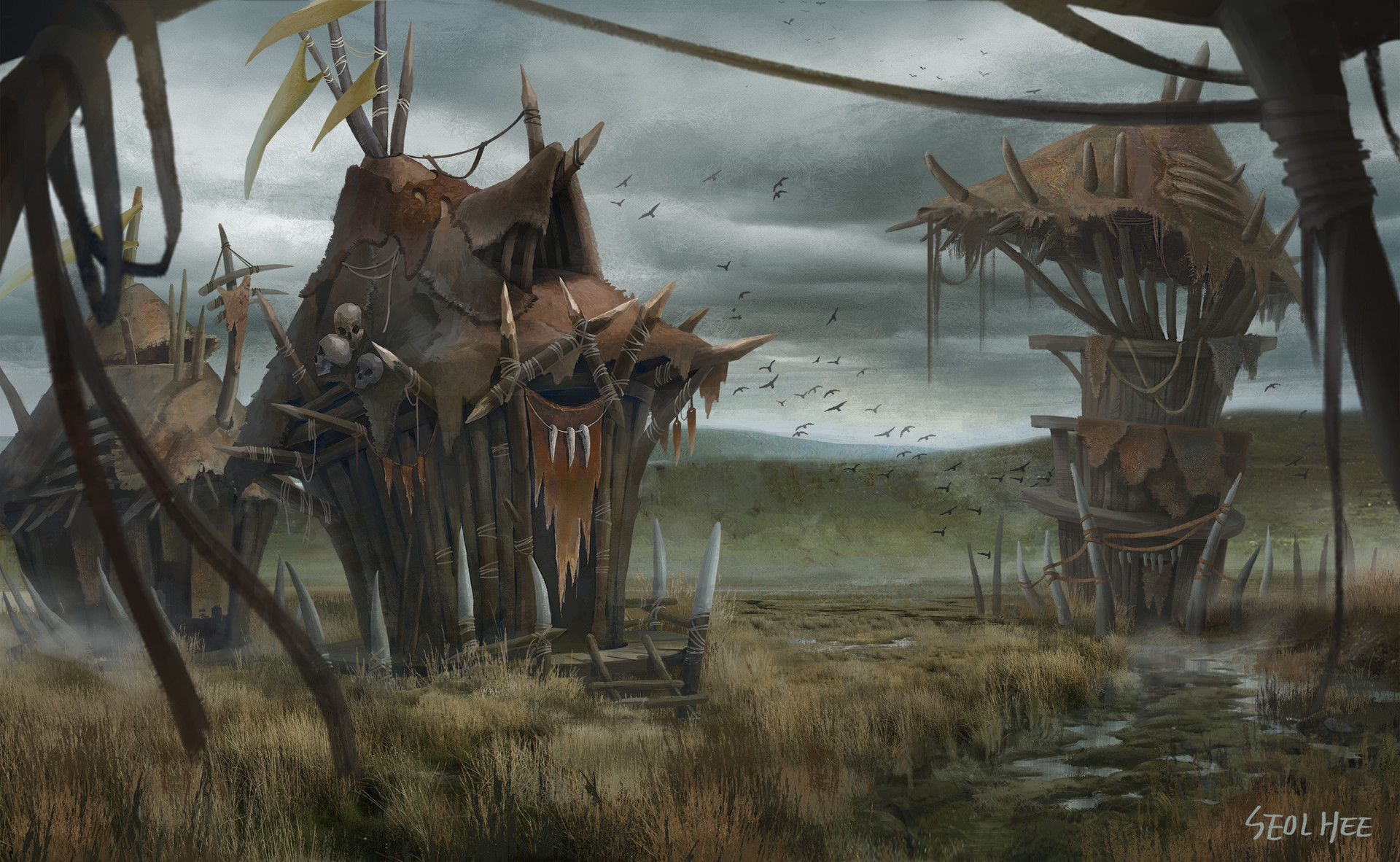This digitally rendered artwork by Seol Hee, displayed on a horizontally oriented canvas, captures a desolate evening scene with a gray, cloudy sky. Three off-kilter, man-made shacks occupy the center of the composition, constructed from hand-carved poles with patched thatch or cloth roofs embellished with spikes and bones. The central shack even appears to have skulls atop it, enhancing the stark and comical nature of the structures. The foreground is dominated by a mix of dried and swampy grassland, showing patches of water and muddy footprints, likely from recent passersby. Additionally, a mountain looms faintly in the distant background, while a flock of birds ascends into the air, adding a sense of movement to the somber, dreary environment. The artist's signature, "Seol Hee," is prominently displayed in the bottom right corner. The predominant colors are brown, gray, beige, black, and white, contributing to the artwork's overall melancholy tone.